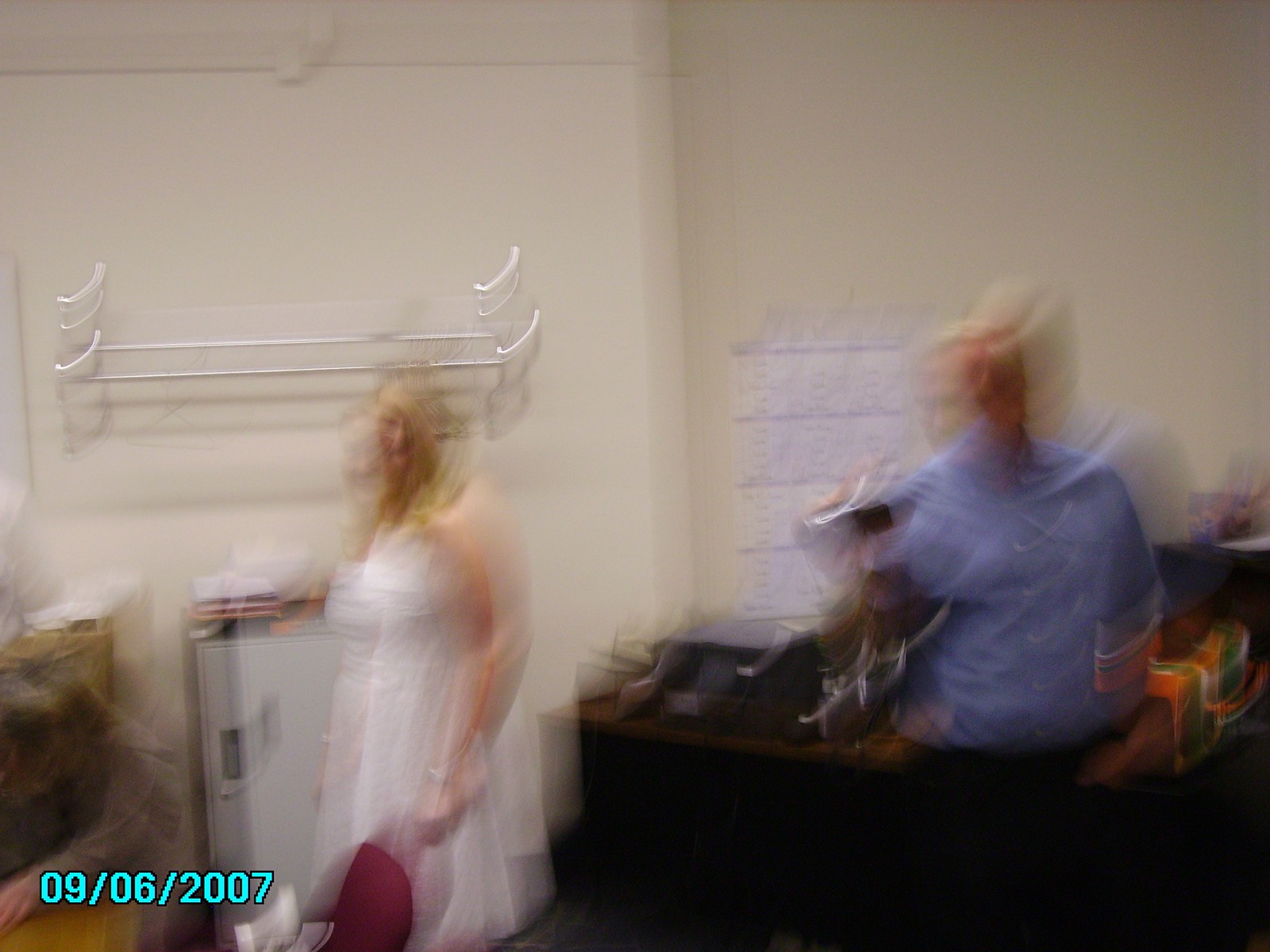In this blurry, out-of-focus photograph dated 09/06/2007, a scene of pre-wedding preparations unfolds. In the bottom left corner, partially visible, is a person getting ready for the big event. Centered prominently and to the right, a larger-sized woman with long blonde hair is dressed in a flowing white wedding gown that ties at the top. She stands in front of a silver metal locker, which is positioned on the floor behind her. Above the locker, a white shelf is mounted on the wall, and further to the right, a paper calendar is affixed to the wall. Below the calendar is a desk with a wood grain top and black metal framing. Standing in front of the desk is a man wearing a short-sleeve blue button-down shirt and black pants; his left hand casually rests in his front pocket.